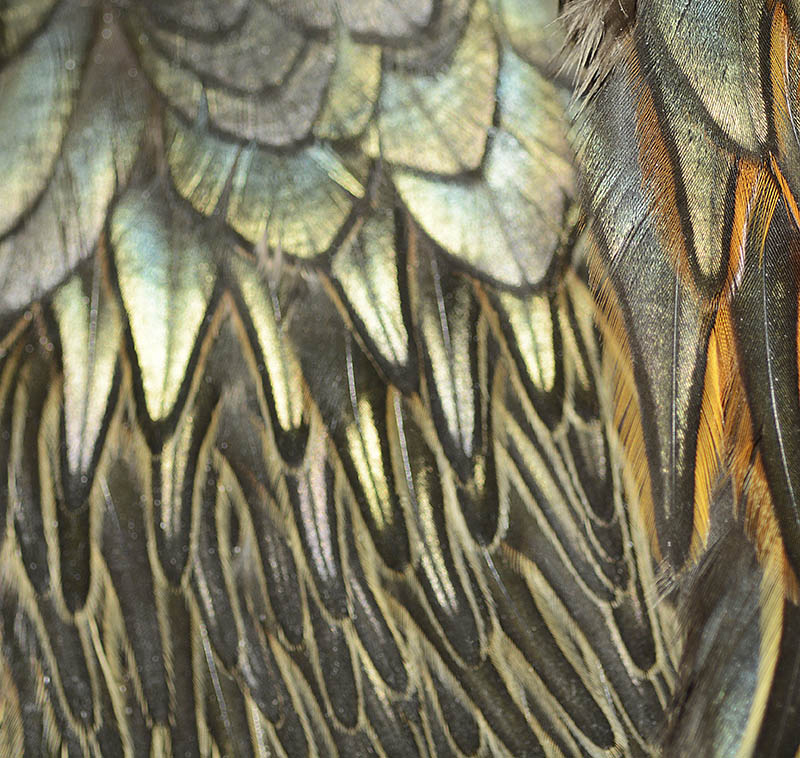The image showcases a close-up view of layered bird feathers, creating a vibrant and detailed pattern. At the top, the feathers are wider with a distinct brown and greenish-blue coloration. As the eye moves downward, the feathers become narrower, longer, and have sharper tips. The feathers in the middle exhibit a greenish-blue hue with black edges, transitioning at the bottom to black feathers with yellow edges. There’s also a variation on the right side of the image, where the feathers start silver at the base, shift to black, and then display orange borders. These feathers are slightly shiny with a dust-like appearance, potentially dandruff. Despite their realistic appearance, the intricate details and bright but dark-tipped colors suggest it might be an artistic representation, possibly part of clothing or jewelry, rather than actual bird feathers.